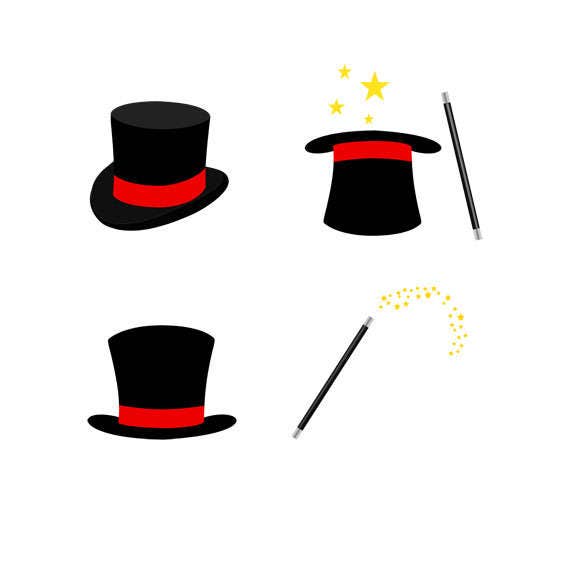This is a detailed cartoon illustration demonstrating a magician's trick in a sequence of four panels against a white background. The first panel presents a black top hat with a red hat band, positioned facing slightly upward at a 45-degree angle. The second panel shows the top hat inverted with its opening facing upward, from which four yellow stars of varying sizes emanate, accompanied by a black magic wand with white ends tilted towards the hat. The third panel depicts the top hat again but from a slightly different angle, right-side up, showcasing the red hat band clearly. The final panel features a black magic wand with white ends, angled at around 50 degrees, emitting a spray of yellowish stars, signifying the activation of the magical effect.